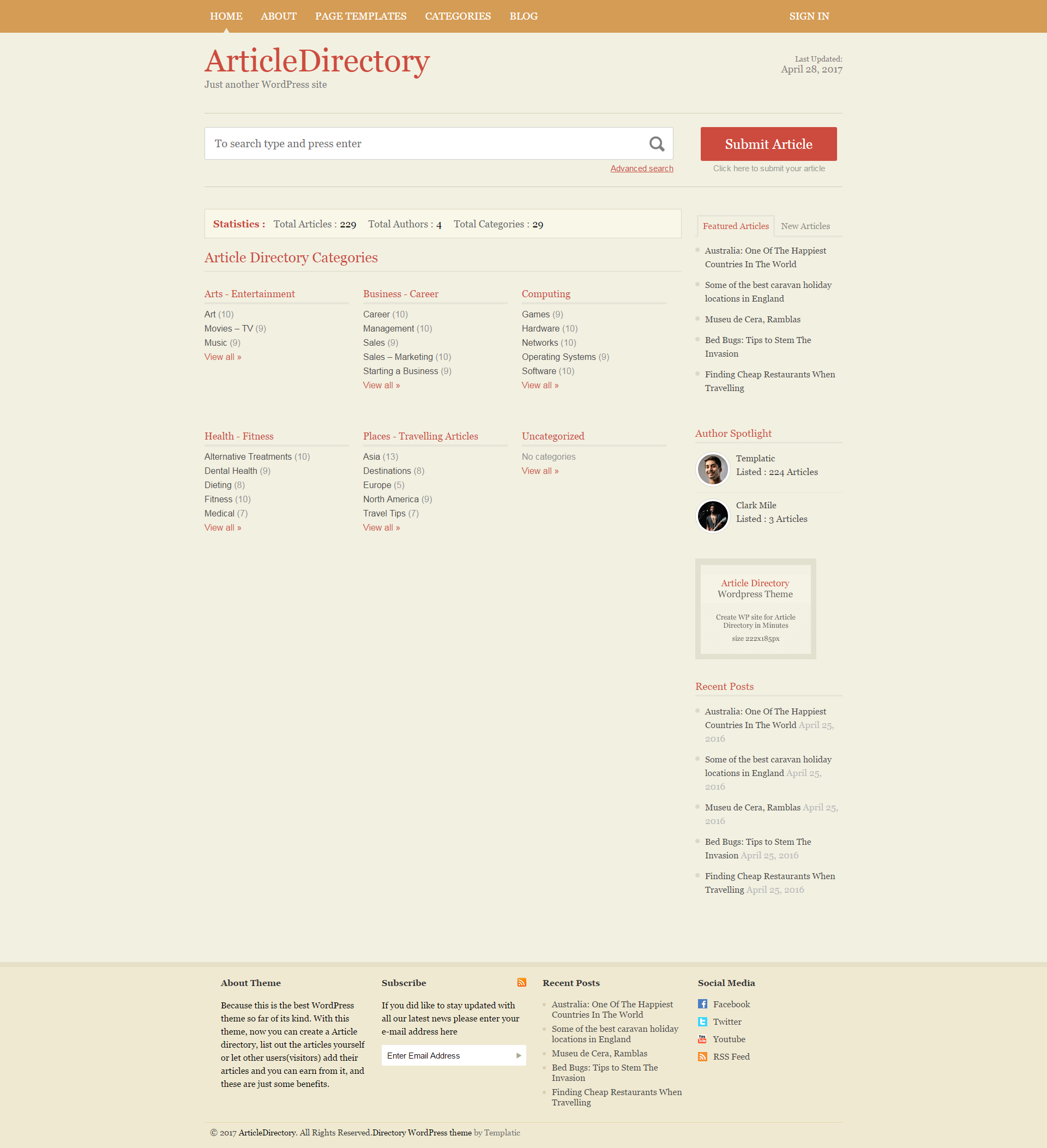The top section of the image features a tab highlighted in a color that is a mix of burnt orange and brown. Inside this tab, the word "Home" is written in white text, accompanied by a triangle, resembling an arrow, pointing towards it. Adjacent to this are other navigation options: "About," "Page Templates," "Categories," and "Blog." On the far right, there is a "Sign In" button.

Below the navigation bar, a row of text in red reads "Article Directory." Underneath, there is a black text that states "Another WordPress Site," followed by an ellipsis and the date "Updated... April 28, 2017."

A horizontal line spans across the width of the page, below which is a white search box outlined in gray. Inside the search box, the placeholder text "Type to search... press enter" is displayed, accompanied by a gray magnifying glass icon. Next to the search box, there is a red rectangle with white text that reads "Subject Article." Below this, the word "Advanced Search" is underlined.

In gray text, there is an invitation to "Click here to submit your article," followed by "Statistics" in red. The statistics are listed in black text: "Total Articles: 229," "Total Authors: 4," and "Total Categories: 29."

Further down, another red heading reads "Article Directory Categories." The categories are listed as follows, in red text:
- Arts
- Entertainment
- Business
- Center
- Computing
- Health and Fitness
- Places
- Travel
- Articles (Uncategorized)

At the bottom of the image, a section highlights authors with an "Author Spotlight." The first author, "Templatic," has listed 224 articles, while the second author, "Clock Mile," has listed 3 articles. The final section advertises an "Article Directory WordPress Theme," with a tagline that suggests creating a website for an article directory in just minutes, though some text is unclear.